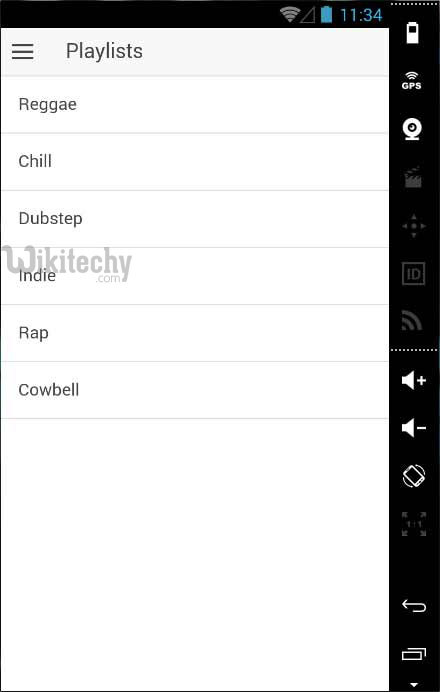The image is a screenshot from a mobile device or possibly an emulator of a mobile device running Android. The interface elements on the right side of the screenshot suggest it's an emulator, as they are vertically stacked icons typically associated with emulator tools rather than a physical device. These icons include GPS, volume controls (plus and minus), a screen rotation option, a back button, and additional emulator-specific controls. 

Focusing on the mobile device's interface, the battery status is shown as fully charged, and the current time displayed is 11:34. Below the time, there is a navigation element labeled "Playlists," accompanied by a menu button represented by three horizontal lines. The app interface has a clean, white background with a list of music genres: Reggae, Chill, Dubstep, Indie, Rap, and Cowbell. Notably, there is a watermark overlaid near the "Indie" option, indicating the source as "wikiteky.com". The lower part of the screen features some white space, which might be reserved for additional content or controls not visible in the screenshot.

Detailed Description:
- **Emulator Tools:** Right side, vertical stack (GPS, Volume +/-, Rotation, Back, etc.)
- **Device Status:** Full battery
- **Time:** 11:34 AM/PM
- **Navigation and Menu:** Playlists label and three-line menu icon
- **Background and Options:** White background with genre options (Reggae, Chill, Dubstep, Indie, Rap, Cowbell)
- **Watermark:** Near "Indie" genre, "wikiteky.com"
- **White Space:** Bottom area of the screen

This descriptive caption encapsulates the key elements and their arrangement within the screenshot.